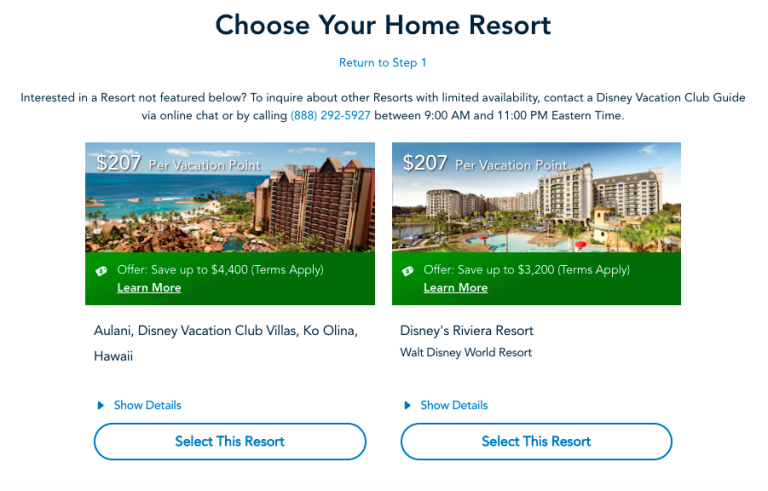Screenshot of Disney Resort Website for Vacation Options

The screenshot depicts a webpage dedicated to selecting a Disney resort, central to the Disney Vacation Club offerings. The header prominently requests visitors to "Choose Your Home Resort," providing two distinct resort options with detailed visuals and information.

At the top of the page, there's a prompt encouraging interested individuals to "choose a resort" by exploring features listed below. Users are advised to contact a Disney Vacation Club guide to inquire about limited availability, either via an online form or by calling the provided phone number. The contact hours are specified as 9 a.m. to 11 p.m. Eastern Standard Time. The guiding text is highlighted in blue for emphasis.

Below this introductory text, two resort options are showcased:

1. **Disney Riviera Resort:**
   - **Offer:** $207 vacation points starting at $4,000 (Terms apply).
   - **Visuals:** The resort features tall brown buildings set against a picturesque blue background. Adjacent to the buildings, there appears to be a beach area.
   - **Additional Details:** A green bar with white text is situated beneath the image, which users can click to learn more.

2. **Disney’s Aulani Resort in Ko Olina, Hawaii:**
   - **Offer:** Also available for $207 vacation points.
   - **Visuals:** This resort displays an image of tall buildings next to a large, inviting pool area.
   - **Additional Details:** Similar to the Riviera resort, a green bar with white text is positioned below the photograph.

Each resort option has an interactive element. Users can click on a link to see more detailed information about the resorts or select the white button with blue text labeled "Choose Resort." 

The page is structured to provide a streamlined and user-friendly experience for prospective guests, clearly outlining options for either the tropical Disney Aulani Resort in Hawaii or the sophisticated Disney Riviera Resort. Both options are priced at $207 per day. The overall layout and design make the selection process straightforward and informative, catering to potential vacation club members.